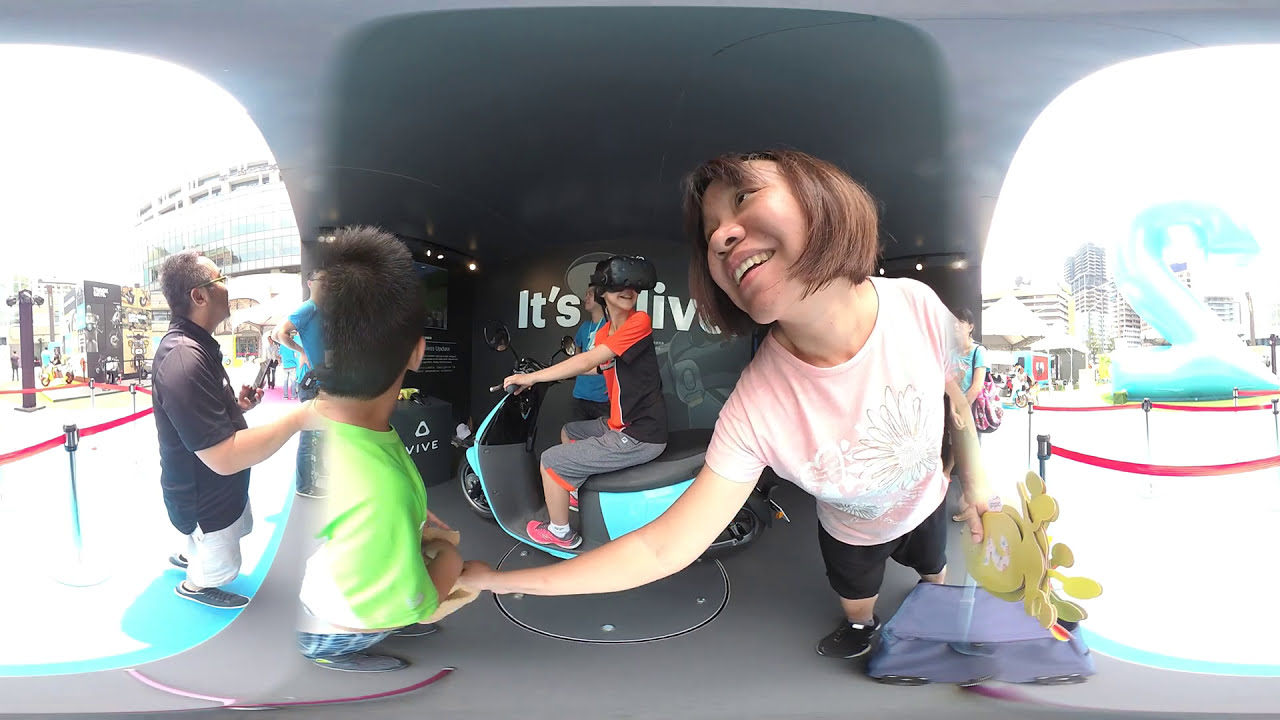In this lively and detailed photograph, a family is enjoying a day at an outdoor amusement park, specifically in a mobile gaming area during daylight. The central focus is on a little boy who is joyfully riding a blue demonstration scooter while wearing a virtual reality headset. His bright neon green shirt and blue shorts make him stand out. He is looking to the side with a broad smile. Behind him, an attendant wearing a blue shirt watches over the scooter. The setup is framed by screens, including one that partially displays the word "LIVE."

The scene reveals an interactive ride area, surrounded by a red rope barrier typical of queuing lines. On the left side of the picture, a man stands outside in the sunlight. Towards the right, part of a large inflatable blue balloon shaped like the number two is visible. 

The family members are actively engaged in the moment. The mother, an Asian woman with short brown hair cut to her chin, is dressed in a pink t-shirt with a silver flower embroidery and black shorts that extend past her knees. She stands close to the boy on the scooter, holding another child in a green shirt, who appears to be watching his brother with fascination. She also has a bag and some sort of craft work in her hands. 

The father, laughing and clearly enjoying watching his son, stands in front of the scooter, adding to the joyful atmosphere. The entire setup hints at a 360-degree immersive experience bringing virtual reality into the real world for an unforgettable family adventure.